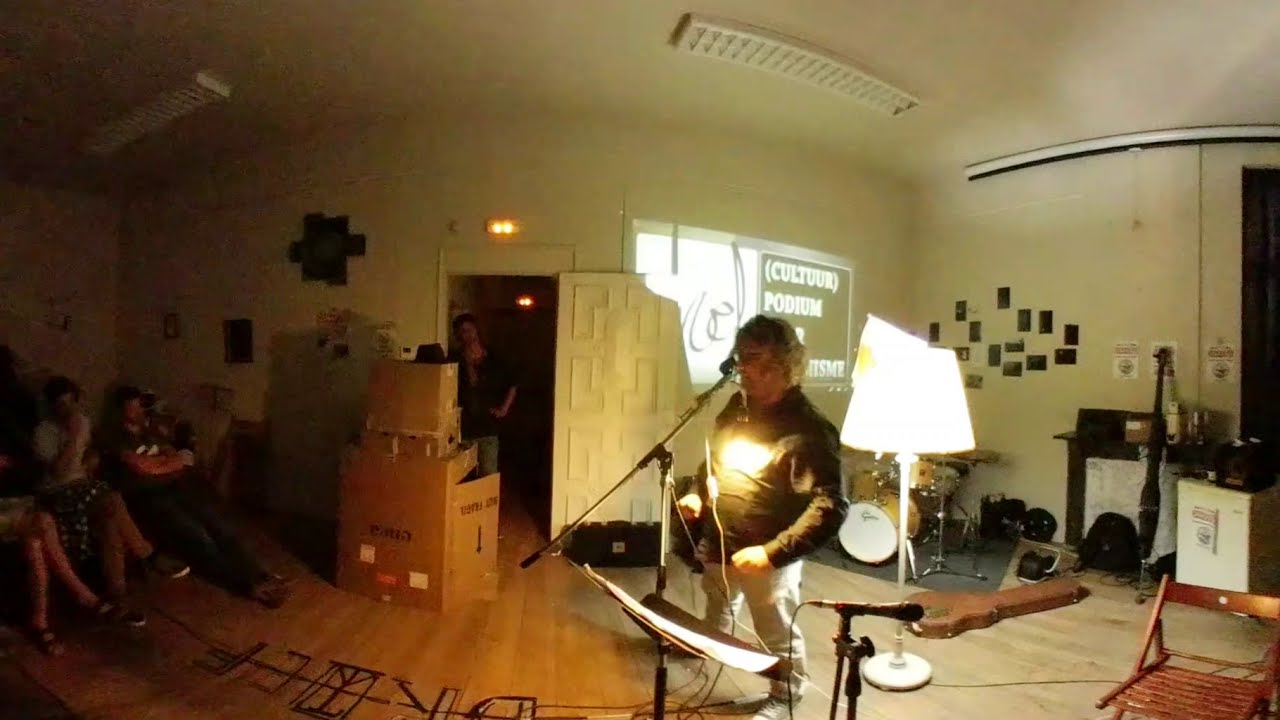In the photograph, an older man with curly grayish hair stands in a cozy living room, doubling as an impromptu performance space, wearing a brown long-sleeved shirt and light khaki pants. Positioned in front of a standing microphone, he is immersed in his music, evidenced by the music stand with papers beside him. Behind him, a large lamp brightly illuminates the scene while the rest of the room remains dimly lit.

The setting is homey, featuring white walls adorned with pictures and photographs, a hardwood floor, and various musical instruments such as a drum set and a couple of amplifiers, though no one else is playing any instruments. To the left, three people are seated on chairs, likely friends or family, appearing somewhat disinterested with one man crossing his arms in a judgmental pose while two women sit with their legs crossed.

The room's small, intimate nature is accentuated by the presence of another observer standing in an open doorway directly facing the performer. Additionally, a subtle projection on the wall behind the musician reads "culture podium," hinting at the informal yet culturally rich atmosphere of the mini concert.